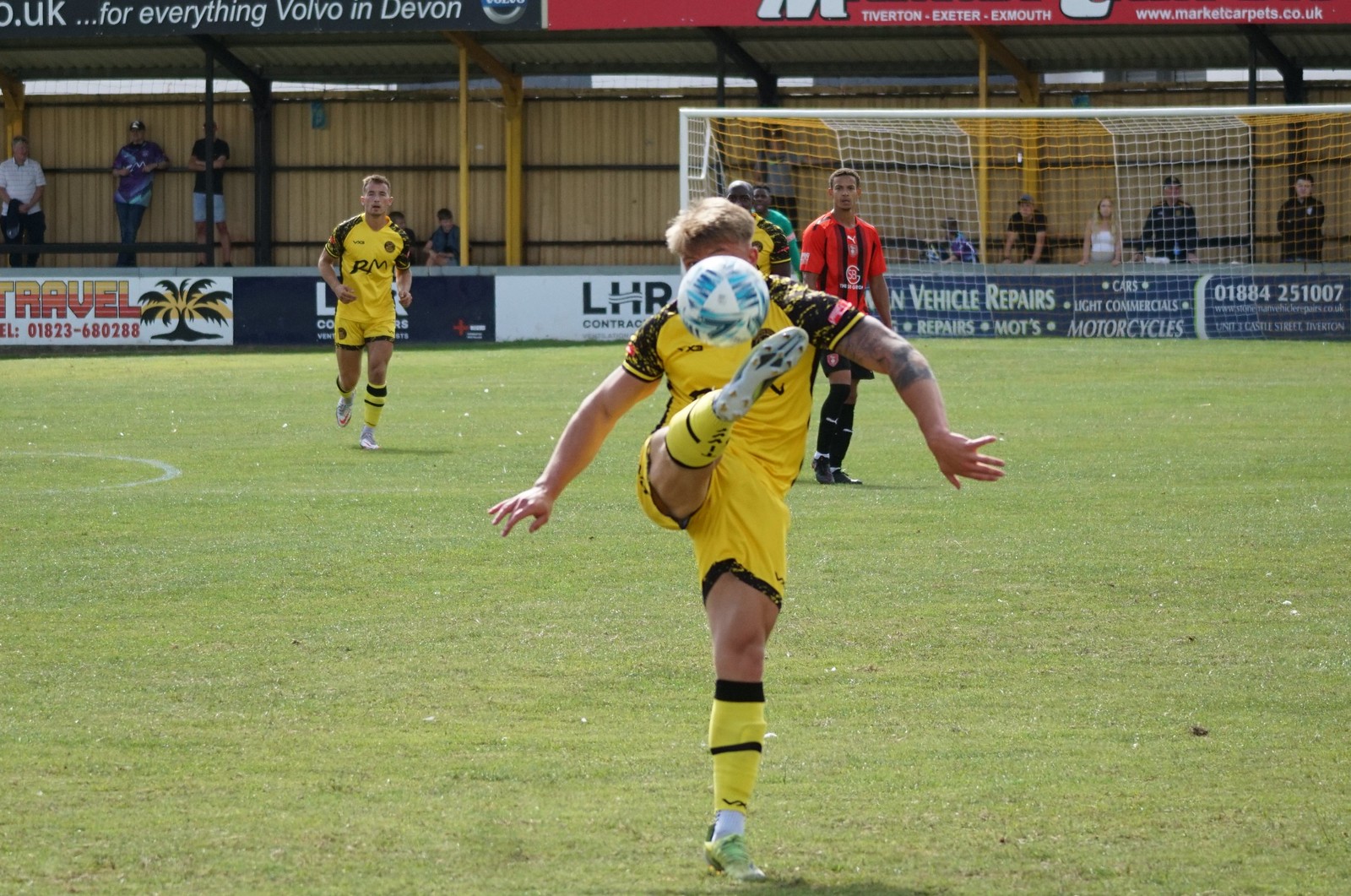In this detailed photograph of a men's soccer game, the central focus is on a player from the yellow team mid-kick, wearing a complete yellow uniform consisting of a short-sleeved shirt, shorts, and socks with black trim. His left leg is raised high, just about to contact the ball, which hovers inches above his foot, obscuring his face. This player also sports noticeable tattoos on his left arm. The backdrop includes the soccer goal stretching from the center to the right side of the image. To the left and behind the central player, two other players in yellow uniforms can be seen, one approaching the kicker. Additionally, a player from the opposing team wearing a light red shirt and black shorts with black socks stands nearby, watching the action. In the far background, there is a short wall adorned with advertisements, behind which various spectators are standing. The grass field is vibrant green, and although the sky is not visible in the cropped frame, the setting is under an open sky. A covered shed-like structure is also present in the background, contributing to the overall scene of an active soccer match.